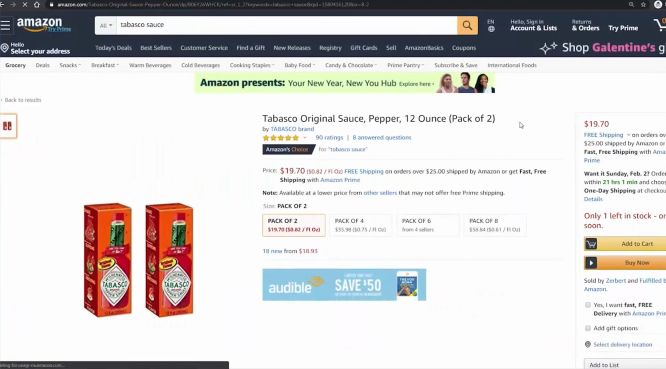This image depicts the Amazon.com webpage displaying the product listing for "Tabasco Original Pepper Sauce" in a 12-ounce bottle, sold in a pack of two. The familiar Amazon logo is positioned on the top left, accompanied by the site's traditional navigation elements including a hamburger menu, a search bar with "Tabasco sauce" entered, and tabs for "Account & Lists," "Orders," and "Try Prime." Beneath these elements, the main section features a detailed product image: two orange boxes each containing a bottle of the famous red pepper sauce. The item is labeled "Tabasco Original Sauce, Pepper, 12 ounce, Pack of Two," and prominently shows a customer rating of approximately 4.5 out of 5 stars based on 90 reviews. The price is listed as $19.70. Purchase options include various pack sizes (two, four, six, and eight bottles), with an "Add to Cart" button situated on the right. The webpage emphasizes urgency with a note indicating that only one unit is left in stock, urging customers to place their orders promptly.